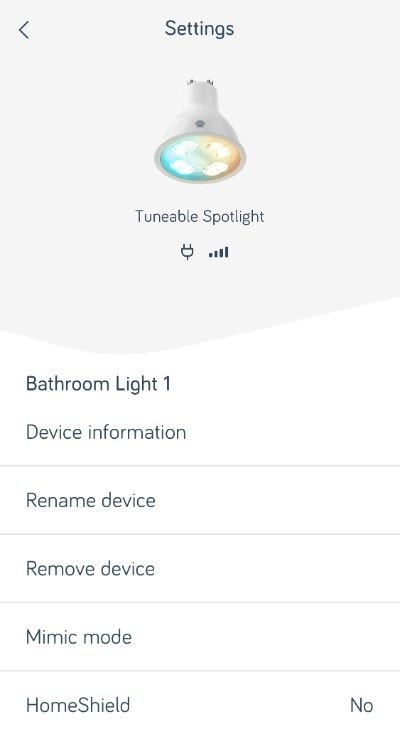The image features a screenshot with a background transitioning from light gray at the top to an angular bottom edge. At the top left corner, there is a less dense arrow symbol pointing to the left. To the right of this arrow, the word "Settings" is displayed. Below "Settings," there is an image of a spotlight with a white casing and a yellowish-blue bulb. Beneath this image, the text "Tunable Spotlight" is shown, accompanied by icons for a plug and a signal strength indicator with four bars.

The section below the gray background features a white backdrop. In this section, black text reads "Bathroom Light 1," followed by "Device Information." A light gray horizontal line separates the subsequent options, which include "Rename Device," "Remove Device," "Mimic Mode," and "Home Shield." On the far right side, there is an indication that says "No."